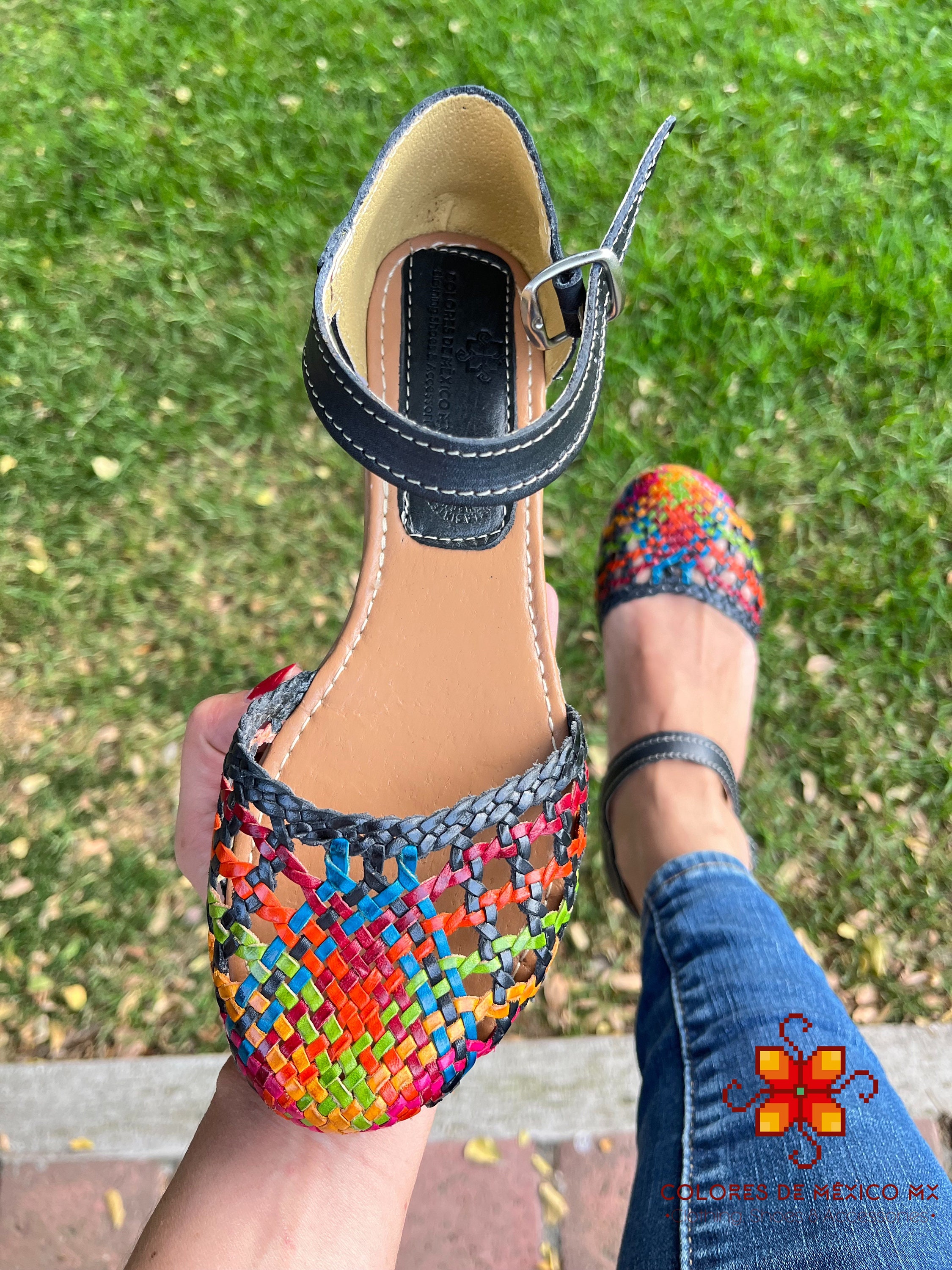In this portrait-oriented photograph, a detailed scene unfolds where a Caucasian woman showcases a colorful sandal. The image is primarily focused on the shoe, which she holds at the toe, revealing the tan-colored sole and a black ankle strap with a metal buckle. The front of the sandal features an intricate woven design with interlocking strips in a rainbow of colors including yellow, green, blue, red, and black. The woman's right leg, clad in tight, skinny jeans, extends to the right side of the image, wearing the matching sandal. Her left hand, with nails painted red, grips the sandal, obscuring part of her palm. The background features a patch of green grass and a curb, hinting at an outdoor setting, possibly a porch overlooking a yard. Additionally, there is a logo in the bottom right corner, depicting a red, orange, and yellow flower with the text "Colores de Mexico MX."